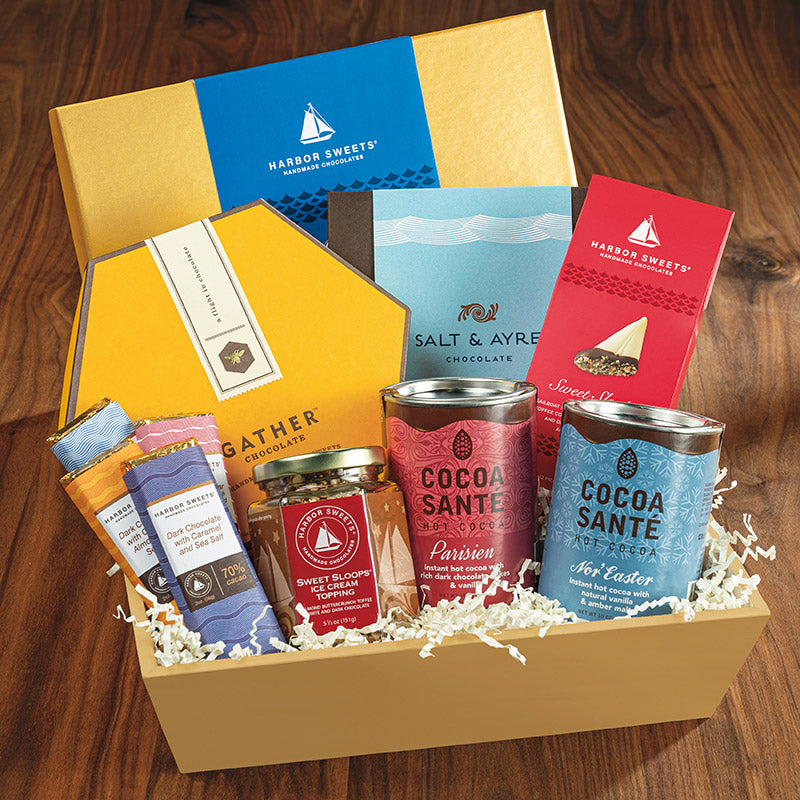A delightful gift box filled with assorted chocolates and cocoa mix treats is showcased on a newish wooden table. The yellow box, adorned with a Harbor Sweets Homemade Chocolates logo featuring a white sailboat against a light blue background with dark waves, contains a variety of sweet items nestled in crinkly white tissue paper. 

At the left of the box, there's a six-sided gold box with a silver lining labeled "A Flight of Chocolate, Gather Chocolate." In the center stands the "Salt and Ayre Chocolate," a light blue box wrapped with a white ribbon and flanked by brown boundaries. On the right side is "Harbor Sweets Handmade Chocolates," a red triangular sweet reminiscent of a fortune cookie, emblazoned with a sailboat and waves motif.

Beneath these, a section of chocolate bars includes options like Dark Chocolate with Caramel Sea Salt (70% cocoa), all from Harbor Sweets. Nearby, a glass jar labeled "Sweet Sloops Ice Cream Topping" promises a delightful addition to any sundae. Completing this sweet assortment, there are two tins of Coco Sante Hot Cocoa mixes: "Parisian Instant Hot Cocoa with Rich Deep Chocolate and Vanilla" and "Nor'east Instant Hot Cocoa with Natural Vanilla and Amber Malt." This curated selection of delectable treats makes an ideal gift for any chocolate lover.